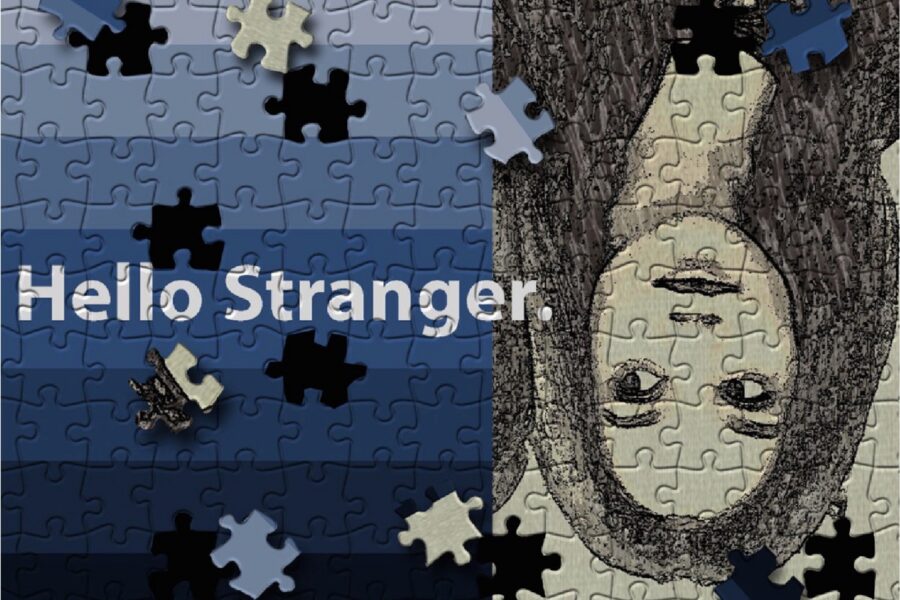This image features a large jigsaw puzzle occupying the entire frame, seemingly blending aspects of two different photographs. The left side displays a gradient of various blue shades, transitioning from a dark blue at the bottom to a bright, almost white hue at the top. Several pieces are missing from this section, scattered across the image. In the center-left, the phrase "hello stranger" is written in white text, partially extending into the right side of the puzzle. The right side depicts an upside-down, hand-drawn image of a woman, with details such as long hair, eyebrows, eyes, nose, and mouth clearly visible. This side also has a white background with missing pieces that have intermingled with those from the blue side. The overall composition suggests the style of a puzzle in progress, with the intriguing mix of colors and elements creating a visually captivating scene.